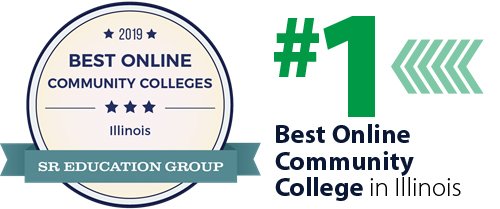A detailed award emblem featured on a white background. On the left side, there is a circular emblem with a black border and an adjacent inner gray circle. Inside the circle, a black star is printed at the top and bottom, flanking the text "2019". In capital letters between the stars, it reads "Best Online Community Colleges". Below this, there are three small stars, bordered by horizontal lines on either side. Underneath the stars, the text "Illinois" is prominently displayed. A grayish-blue ribbon at the bottom of the emblem reads "SR Education Group". 

To the right of the circle, the award message continues with large green text displaying "#1", followed by a series of light-blue arrows formed by less-than symbols, pointing right. Below this, "Best Community College" is written in black text, with the phrase "In Illinois" appearing in gray text beneath it. The rest of the image contains empty white space, keeping the focus on the described award.